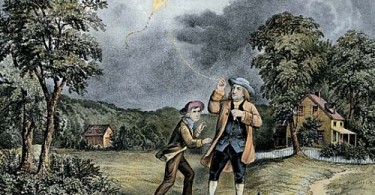This detailed painting, reminiscent of an illustration from Chaucer's days, captures Benjamin Franklin flying a yellow kite in a stormy gray sky, likely during his famous experiment involving electricity. Rendered in an old-fashioned style, possibly an oil painting, it portrays Franklin in a beige coat, knickers, a blue flat hat, and a vest, grasping the kite string with both hands. Beside him stands a young assistant, dressed in a coat, brown pants, and a tipped-up flat hat, seemingly reaching out animatedly, perhaps to take hold of the kite string himself. The duo is set in a grassy meadow, flanked by a small hut to the left and a larger story-and-a-half house with a dormer and porch to the right, surrounded by mature trees and a white picket fence. The landscape features rolling hills and a curving path leading to the right-hand house, evoking a serene rural backdrop to this dynamic scientific endeavor.